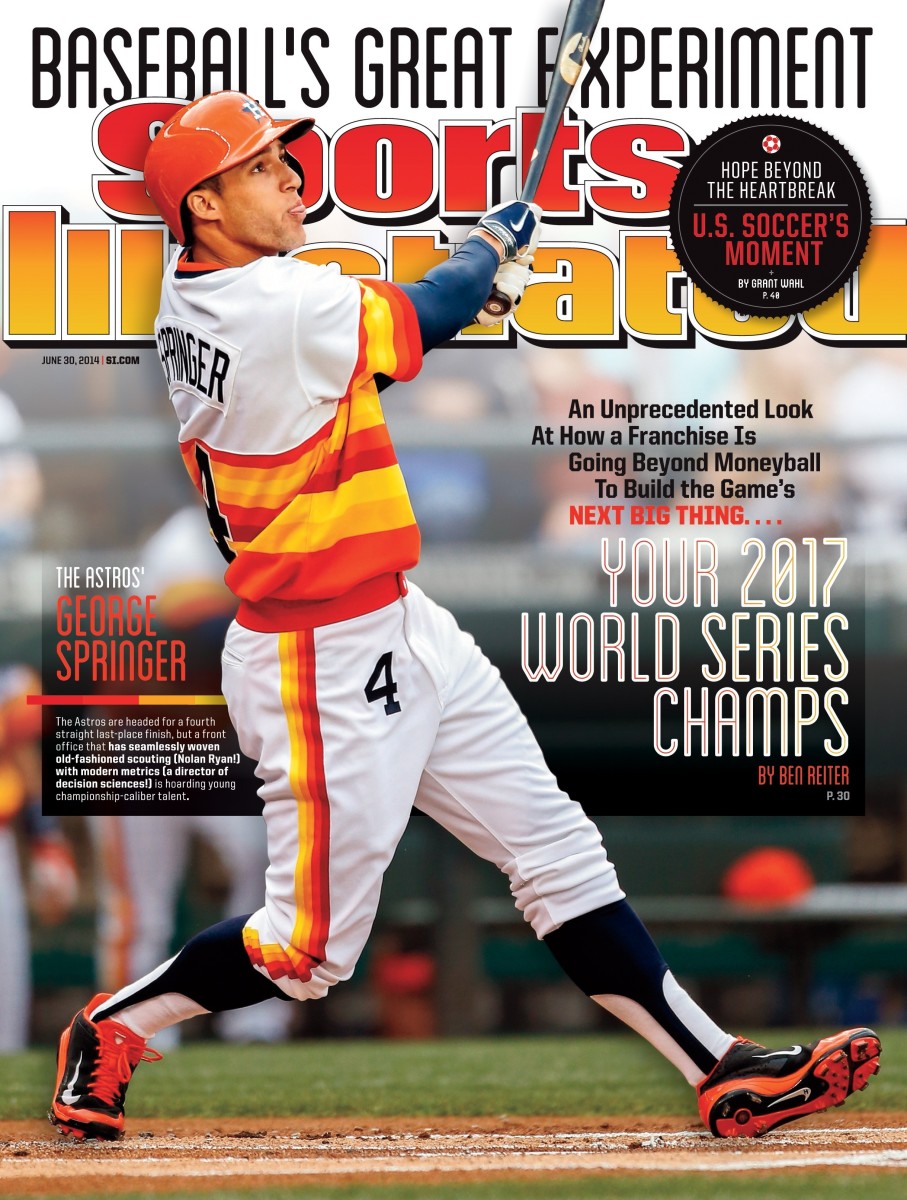The cover of the Sports Illustrated magazine, dated June 30, 2014, prominently features George Springer of the Houston Astros. Titled "Baseball's Greatest Experiment," the cover highlights an in-depth story by Ben Reiter on page 30 about how the Astros franchise is revolutionizing the game beyond the concepts introduced in Moneyball to build a championship team, evidenced by their future 2017 World Series win. Springer, depicted in a dynamic action pose presumably after a powerful swing, dons a colorful jersey in shades of yellow and orange with blue sleeves and white shoulders, white pants, sporty shoes, and a red-orange helmet for protection. The background text emphasizes the team's unique blend of traditional scouting and modern metrics aimed at creating championship-caliber talent, despite being poised for their fourth consecutive last-place finish. Additionally, the cover mentions a feature by Grant Wahl on page 48 about U.S. Soccer titled "Hope Beyond the Heartbreak," nested within a circular badge at the far right.